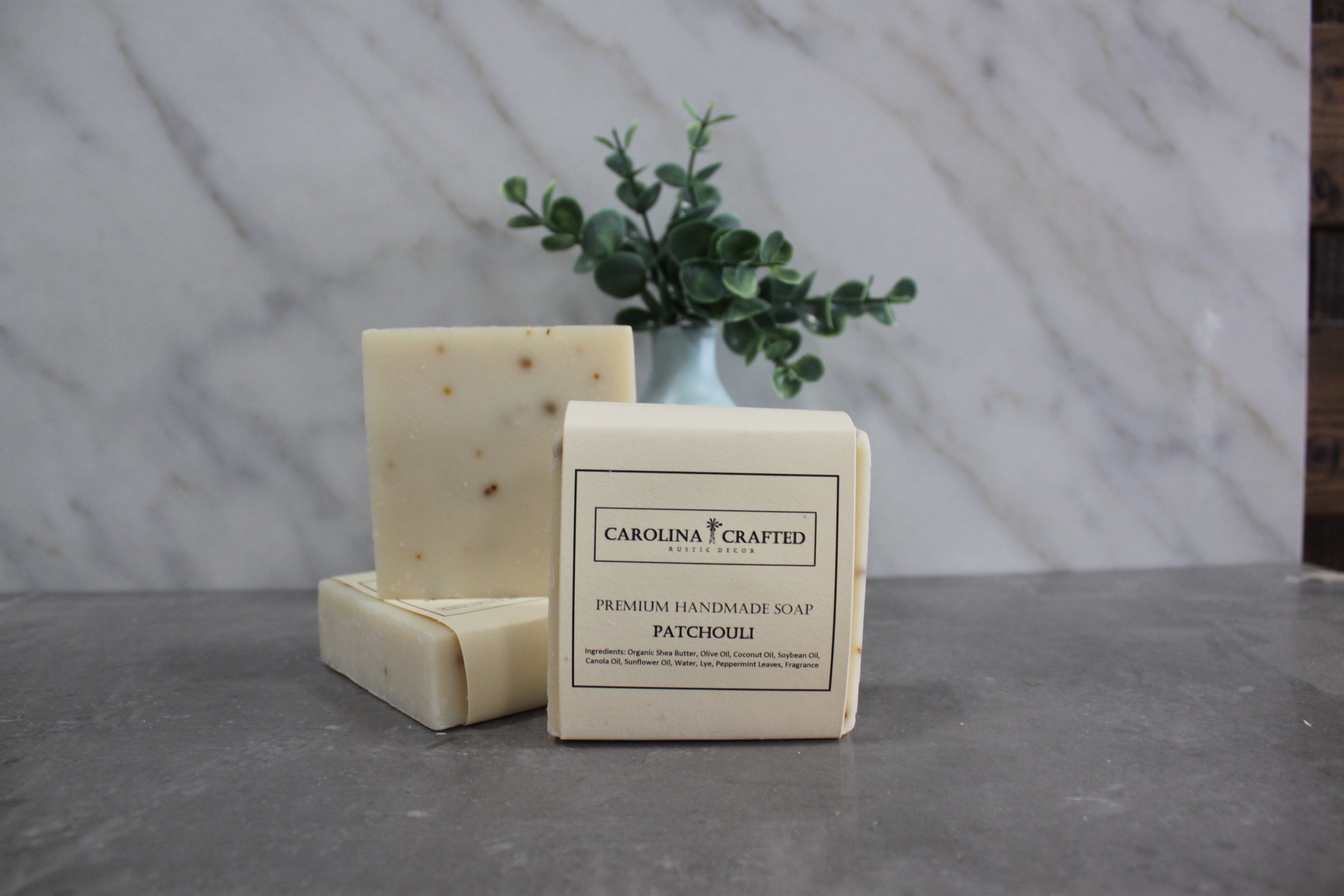This landscape-oriented, color photograph showcases a scene of handcrafted soap bars arranged on a dark gray countertop. The backdrop is a shiny white marble wall with subtle gray streaks, contributing to a clean and elegant aesthetic. The main subject features three bars of soap: the central focus is a standing soap bar, wrapped in off-white, bone-colored packaging. The label prominently displays "Carolina Crafted Rustic Decor" in bold black text, followed by "Premium Handmade Soap" and the scent marker "Patchouli." Behind it, on the left, two more bars of soap are visible—one lying flat and the other stacked upright without packaging, revealing a creamy beige color with dark speckles, reminiscent of pepper jack cheese. Completing the composition, a white vase filled with dark green eucalyptus leaves peeks from behind the soap, adding a touch of natural greenery. The overall style of the image can be described as photographic representationalism, emphasizing realism and meticulous detailing typical of product photography.